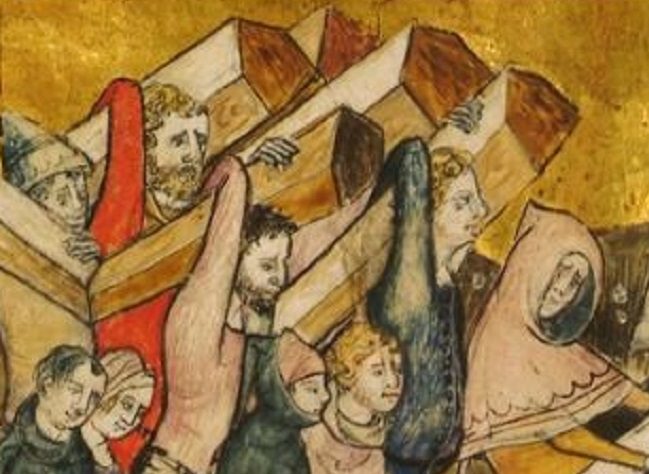This classic painting, reminiscent of an older drawing, portrays a group of people, predominantly men, carrying long, pentagonally-shaped wooden logs on their backs. The characters, visible mostly from the waist up, appear somber and stare seriously ahead, with many looking down. The central figure, distinct in a hooded shawl of tan hue, walks in front without carrying any wood. Behind this person, other individuals persist with their burdens, dressed in blue, pink, and bright red clothing. The background features a yellowish-brown sky, creating a stark contrast with the dark gray field visible on the right side, enhancing the somber mood of the scene.